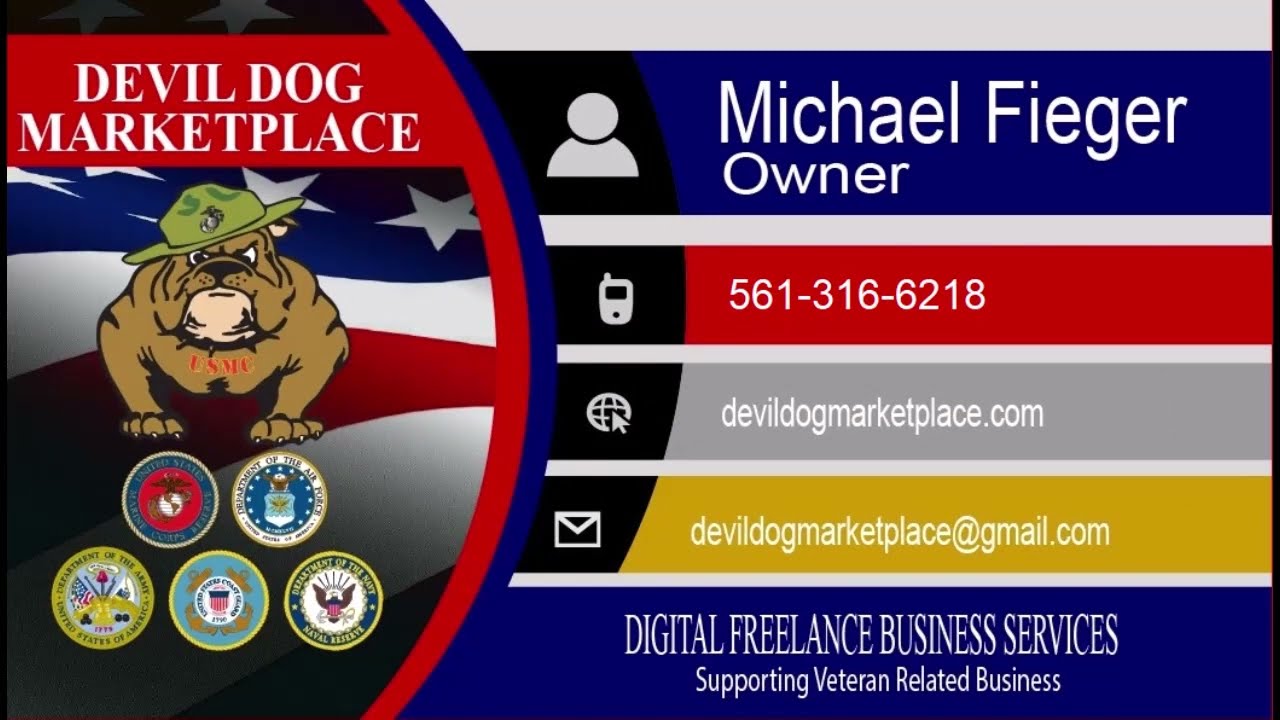This is a color photograph of a business card for Devil Dog Marketplace. The left side features white lettering on a red background at the top, displaying "Devil Dog Marketplace" above a logo of a tough-looking bulldog in a marine drill sergeant hat, set against an American flag with visible stars. Surrounding the bulldog are several military service logos, including those for the Marine Corps and the Department of the Navy.

On the right-hand side of the card, there are bands of blue, red, gray, and mustard colors. At the top, "Michael Feger, Owner" is written in white text on a blue background, accompanied by a gray cartoon figure icon. Below that, a phone number, 561-316-6218, is displayed in white on a red background with a phone icon to its left. The website "devildogmarketplace.com" follows, printed in white on a gray band. Beneath that, the email address "devildogmarketplace@gmail.com" appears in white on a mustard-colored band. At the bottom of the card, in white text on a blue background, the phrase "Digital Freelance Business Services Supporting Veterans-Related Business" is inscribed. 

The card uses various colors such as gray, blue, red, gold, silver, green, and brown, with a strong emphasis on American patriotic colors like red, white, and blue, reflecting its military and veteran-supportive theme.